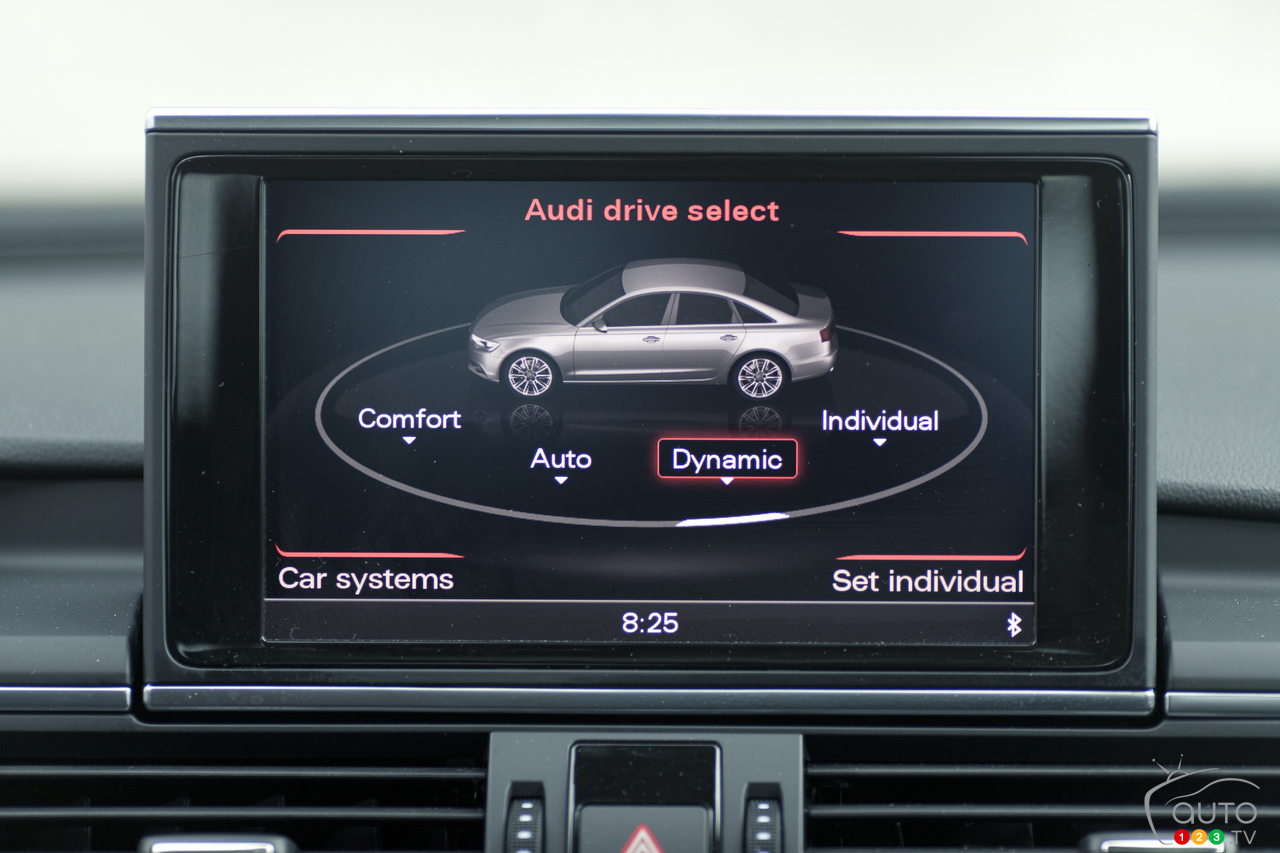The photograph captures the dashboard of an Audi vehicle. Central to the image is the car's integrated GPS and control screen, prominently displaying "Audi Drive Select" at the top. A silver Audi sedan is depicted on a circular platform within the display. The screen features various drive modes: "Comfort," "Auto," "Dynamic" (highlighted with a rectangle indicating selection), and "Individual," each accompanied by a downward arrow. The bottom left of the screen reads "Car Systems," while the bottom right says "Set Individual." Below the screen are the car's air vents and their adjustable controls. The digital clock on the display shows the time as 8:25. The edges of the photograph reveal a glimpse of the outside through a blurred windshield, adding context to the car's interior setting.